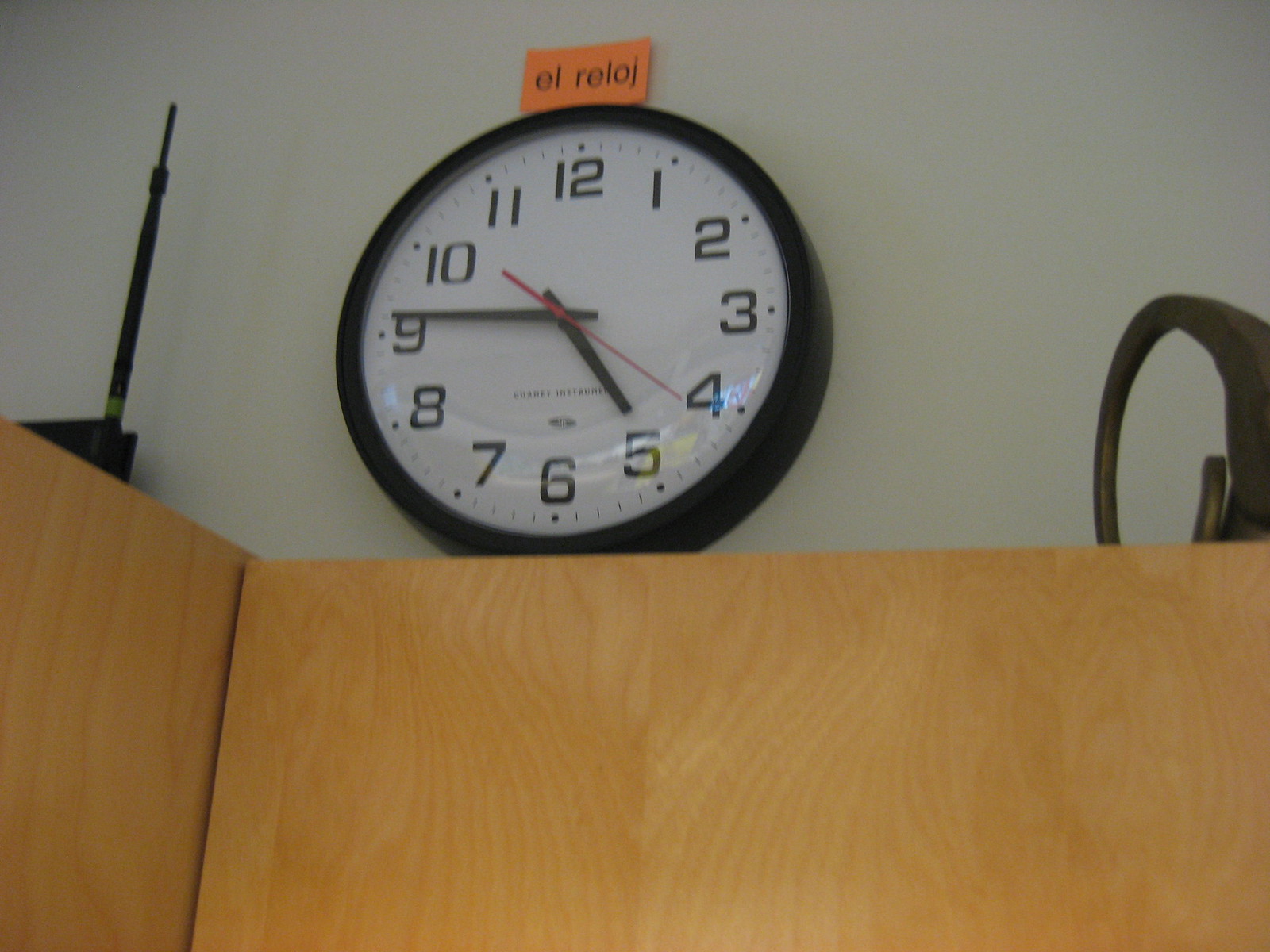A black circular wall clock, presently leaning rather than mounted, sits against a wall. It features a white face with bold, black numerals marking the hours from 12 at the top to 11. The minute and hour hands are black, while the second hand is strikingly red. Although there is a brand name visible on the clock, it remains unreadable due to a blur in the image. Resting atop the clock is a horizontal rectangular piece of orange construction paper with the word "El Reloge"—spelled R-E-L-O-G-E—typed on it. The clock itself is perched on a wooden structure, resembling a desk, which has a blonde oak finish. The desk, or structure, provides a sturdy base against which the clock is propped.